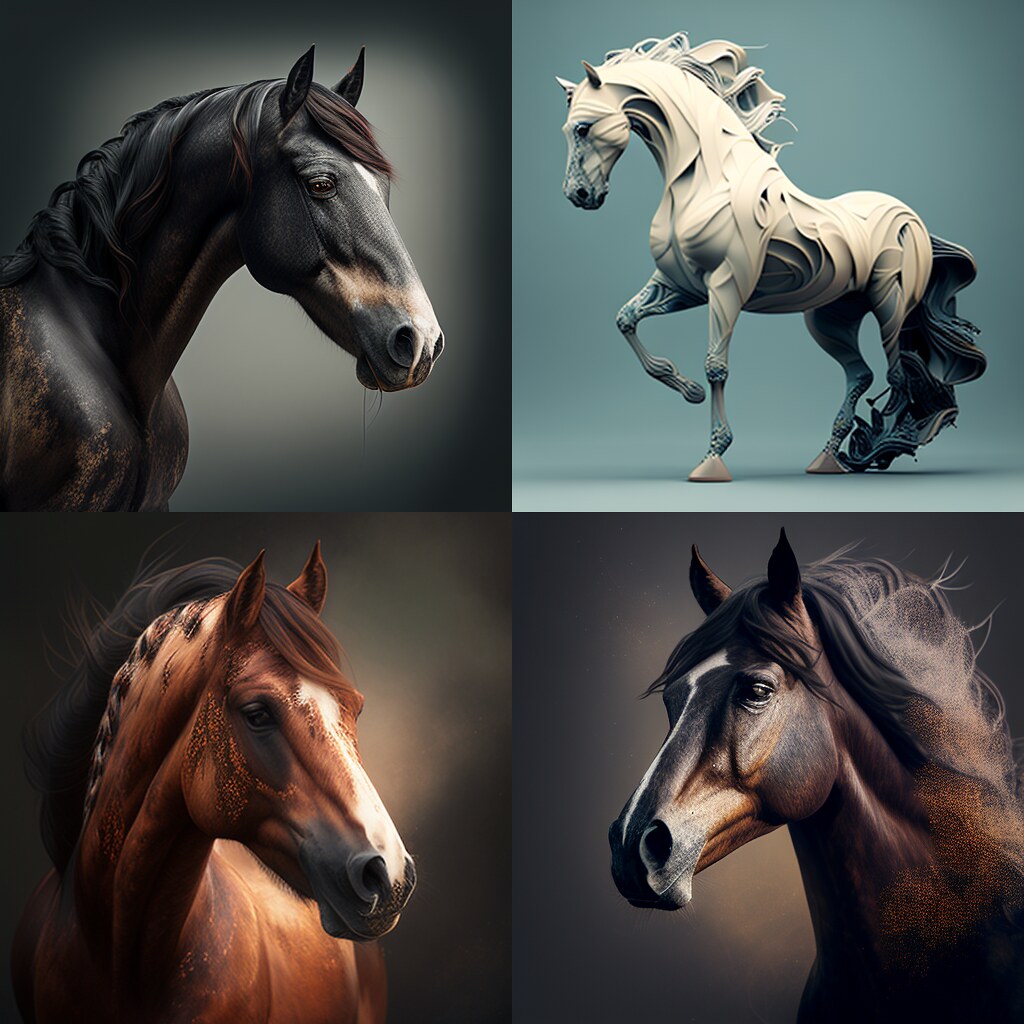The image presents a collection of four computer-generated horse illustrations arranged in a larger square, each showcasing unique design elements and perspectives. 

In the top left quadrant, there is a side perspective of a predominantly black horse with subtle white splotching on its body, a black mane, and light brown markings accentuating its face, running down the nose. The background transitions from dark grey to light grey.

The top right quadrant displays a full-body view of an abstract, white horse rendered with a 3D modeling program, featuring wavy contours and blue-tinted ceramic-like hooves. Its tail is a distinctive, flowing blue, set against a blue backdrop.

In the bottom left quadrant, a frontal view depicts a horse with rich brown fur, a flowing auburn mane, and a prominent white stripe extending from its forehead to the tip of its nose. This horse looks off to the right, with a dark grey background enhancing its features.

Lastly, the bottom right quadrant shows the head and upper torso of a dark brown horse with a white streak down its snout. Its mane is a striking mix of light grey and white. The background transitions from grey to a light purple hue, adding depth to the representation.

Together, these four images create a striking composite of diverse equine artistry.